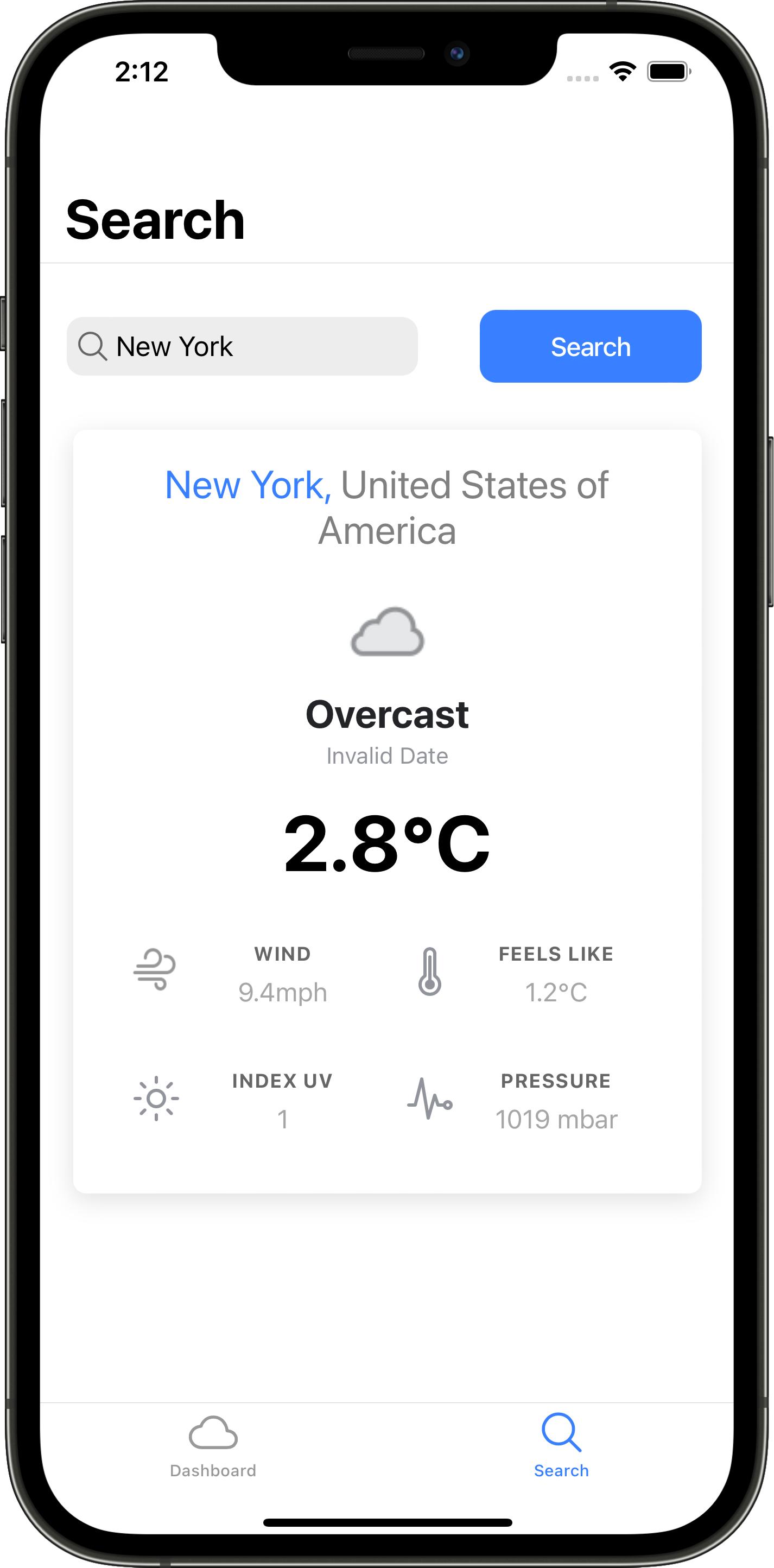The image displays a phone screenshot captured at 2:12, indicated by the time shown. The device has a full battery and a strong Wi-Fi signal, all set against a white background. Prominently displayed at the top in large black bold letters is the word "Search." Directly below is a grey search box containing the text "New York," accompanied by a magnifying glass icon. To the right of this search box is a blue button labeled "Search."

Beneath this section lies a white box with a grey border, featuring weather information for New York. The text "New York" appears in blue, followed by "United States of America" in black. The weather condition is described as "overcast" with an accompanying cloud icon. An "invalid date" marker is present, along with the temperature reading of 2.8 degrees Celsius. A wind icon indicates a wind speed of 9.4 MPH. Additionally, a thermometer icon displays a "feels like" temperature of 1.2 degrees Celsius, and a sun icon indicates a UV index of 1. A line graph symbol conveys the atmospheric pressure reading of 1019 mbar. At the bottom of the screenshot are two buttons: one labeled "Dashboard" and another "Search."